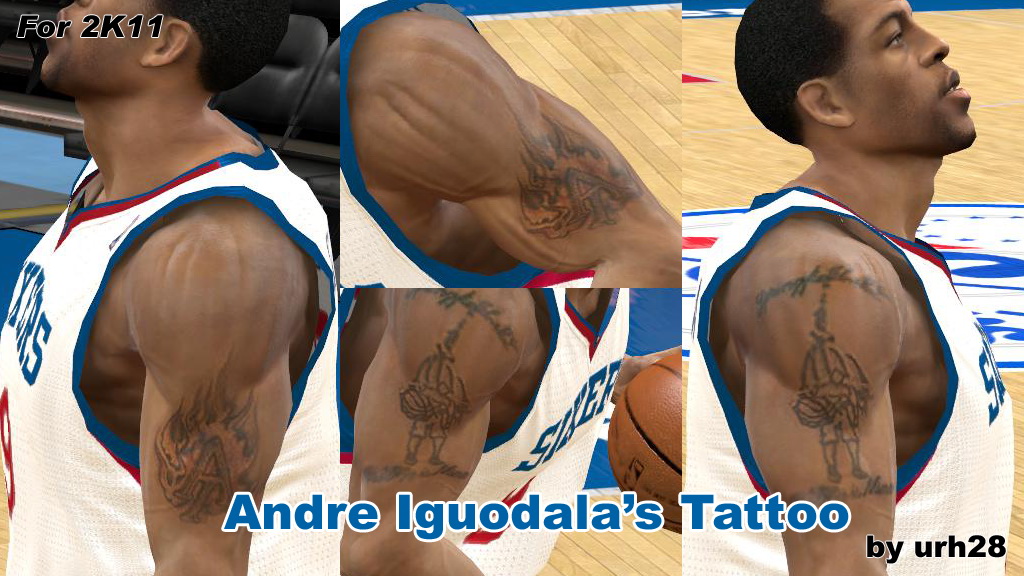This image is a collage consisting of four digitally rendered screenshots, likely from an NBA video game, depicting the basketball player Andre Iguodala and his tattoo. Starting from the left, the first rectangle captures a side profile of Andre from the nose down, showcasing his white sleeveless jersey with "Sixers" printed in blue across the chest. The armholes are outlined in blue, and the V-neck features a cranberry-red trim. Prominently, there is a tattoo on his left upper arm that resembles an "A" with flames behind it. 

The two center photos are arranged vertically. The top center image offers a closer view of the flaming "A" tattoo, highlighting its intricate details. Below it, the second center image reveals a different side of Andre, focusing more on his right arm's tattoo, though it is too blurry to clearly identify. 

On the right side, the larger photo provides a full-view close-up of Andre in action, presumably playing basketball. The right side profile reveals additional details of his jersey and the tattoos. Overlaying these images, in bold blue text, it reads "Andre Iguodala's tattoo," followed by "by URH28" written in black at the bottom.